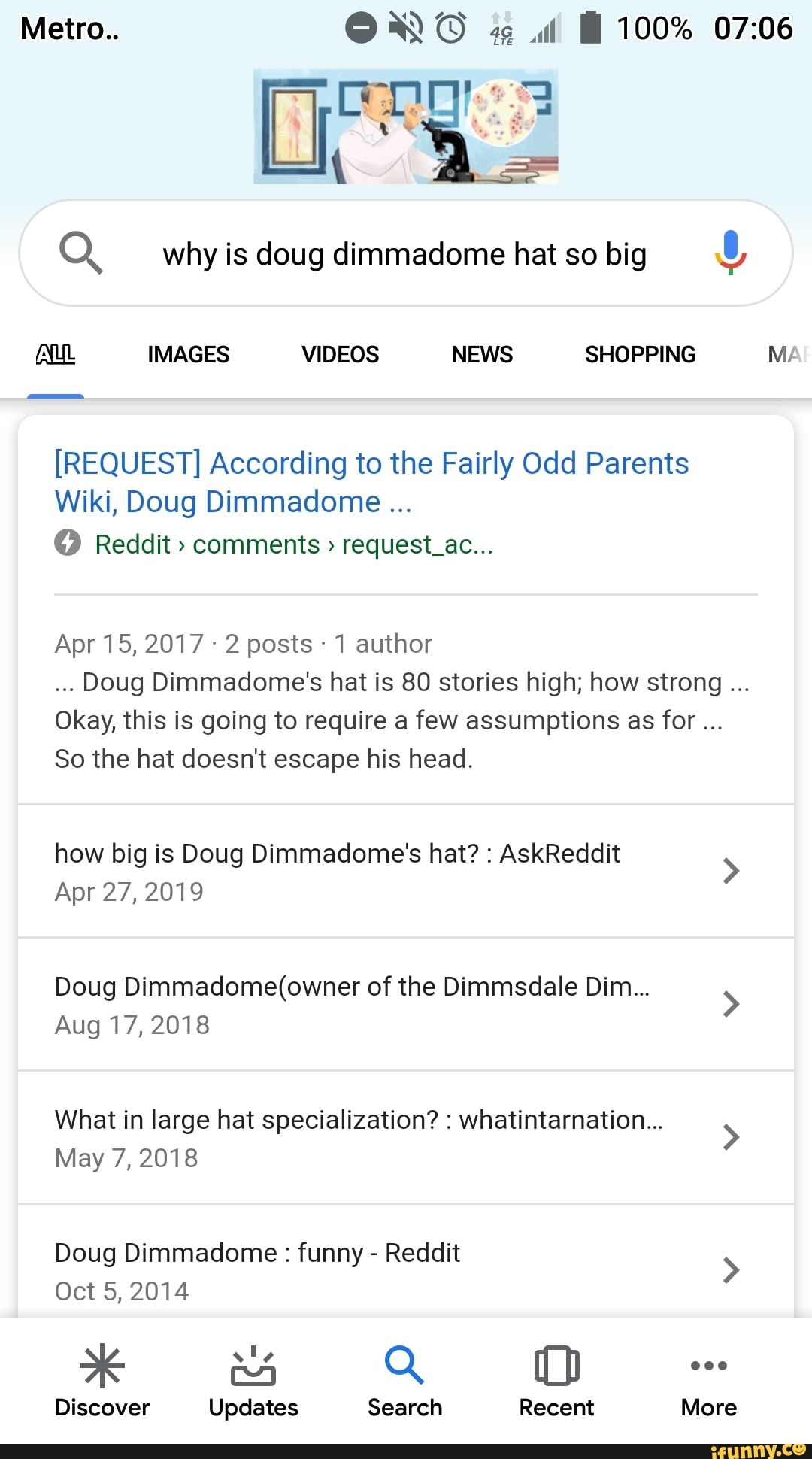**Caption:**

The image shows a smartphone screen, specifically a Metro phone, indicated by the Metro logo in the top left corner. The phone’s status bar displays comprehensive connectivity and system information: a Wi-Fi signal, a muted sound icon, an alarm clock set, 4G network bars, and a fully charged battery. The current time is 7:06.

Centered on the screen is a search query entered into a browser, reading "Who is Doug Demidome? Why is Doug Demidome's hat so big?". Beneath the search bar, a snippet from the Fairly OddParents Wiki provides an initial overview of Doug Demidome, while the following results stem from Reddit discussions. One notable Reddit comment claims that Doug Demidome's hat is 80 stories high, sparking debates about the hat’s enormity and the character's signature look. The Reddit post includes humorous inquiries about the practicality and structural integrity of such an oversized hat, reflecting the quirky fascination with this character from *The Fairly OddParents.*